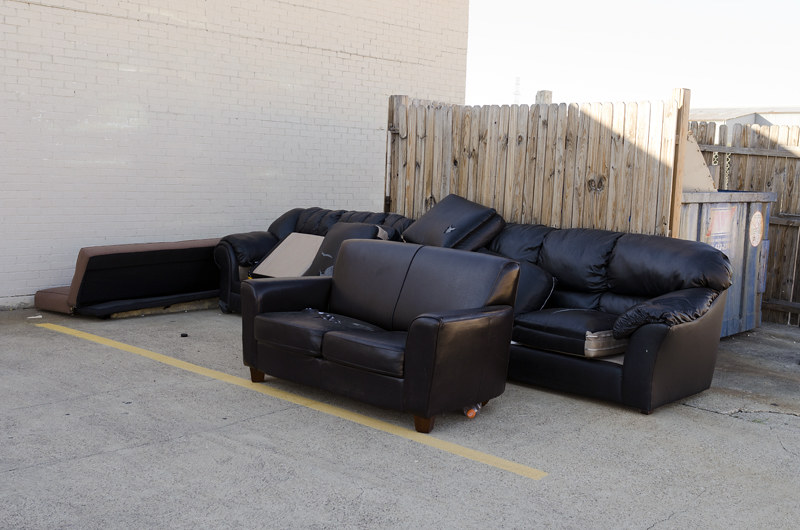This outdoor photograph features a parking lot adjacent to a white-painted brick building. The lot, paved with asphalt, is marked by a prominent yellow line designating parking spaces. Centrally positioned in the image is a fenced enclosure made of wood, containing a large gray trash receptacle filled with what appears to be cardboard. In the foreground and around the parking area, there is a disorganized collection of furniture awaiting disposal. This includes at least four large sofas, primarily made of black imitation leather, with some showing visible wear and tear such as cuts exposing the white interior. A particularly notable detail is a pink sofa lying on its side without visible legs. Also scattered among the furniture are brown couches, including a damaged loveseat displaying cuts and wear. The overall scene conveys a sense of neglect and abandonment, emphasizing the dilapidated condition of the items awaiting removal.